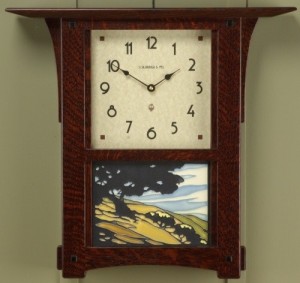The image showcases a wall-mounted wooden clock, crafted in a likely reproduction of the old Craftsman style, featuring a rich cherry wood frame with a dark stain. The clock stands approximately one and a half feet tall by one foot wide, framed by a flattened, flared-out top, reminiscent of a tray or small mantle.

At the upper section of the clock, the face exhibits a simple yet refined Art Deco style, boasting black numbers in a slightly rounded retro font against an off-white background. Currently, the time displayed is 1:50, with the short hand near the 2 and the long hand on the 10.

Beneath the clock face, a stained glass panel captures a tranquil landscape scene. The artwork features a black tree in the foreground, surrounded by black bushes. The serene background showcases a blue sky with white clouds, along with a green and yellow field. This picture is perfectly framed by the reddish-brown cherry wood, providing a warm and elegant contrast.

The entire clock is set against a light dusky green wall, further emphasizing its classic yet timeless appeal.